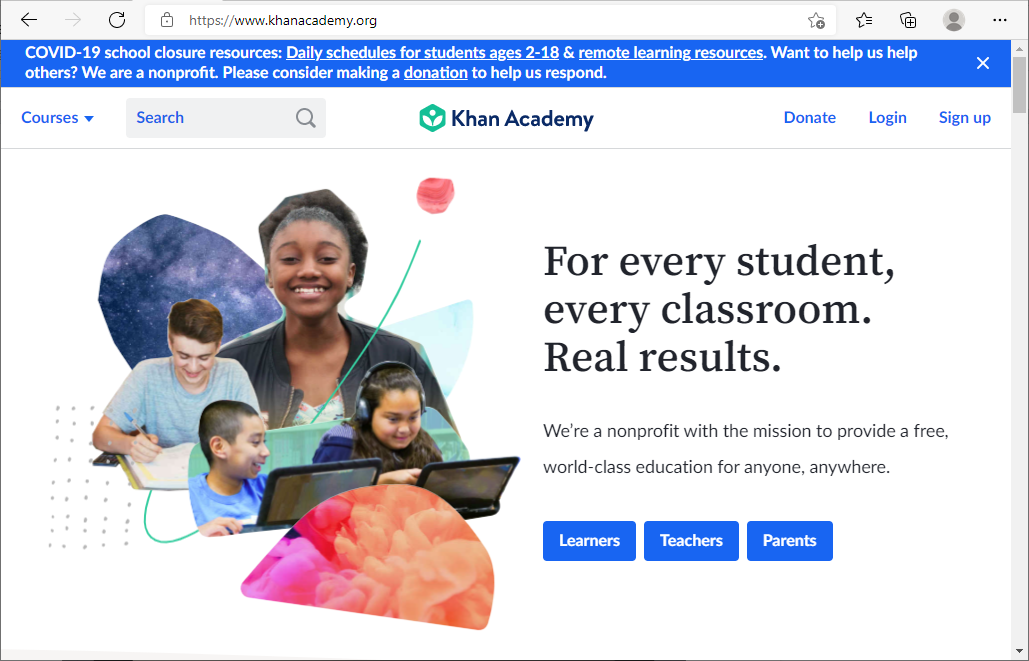The screenshot captures the homepage of Khan Academy's website, identifiable by the domain conacademy.org displayed at the top. A prominent blue banner at the top of the page serves as a notification urging visitors to explore COVID-19 school closure resources and daily schedules for students aged 2-18. It highlights available remote learning resources, emphasizing the non-profit's need for donations to aid in their response efforts. 

Upon dismissing this banner, users can navigate through the website. On the left-hand side, there's a menu labeled "Courses," likely offering access to a wide range of educational materials. Adjacent to it, the Khan Academy logo is prominently displayed, alongside a search bar, and buttons for donations, logins, and sign-ups. Returning users can easily log in or new users can create an account from this section.

The main section of the webpage features an image of students engaged in learning, equipped with laptops, paper, and pencils. Accompanying the image is text that reads, "For every student, every classroom, real results. We are a non-profit with a mission to provide a free, world-class education for anyone, anywhere." Below this mission statement are three blue buttons for different user groups: learners, teachers, and parents, which likely offer tailored resources for each category.